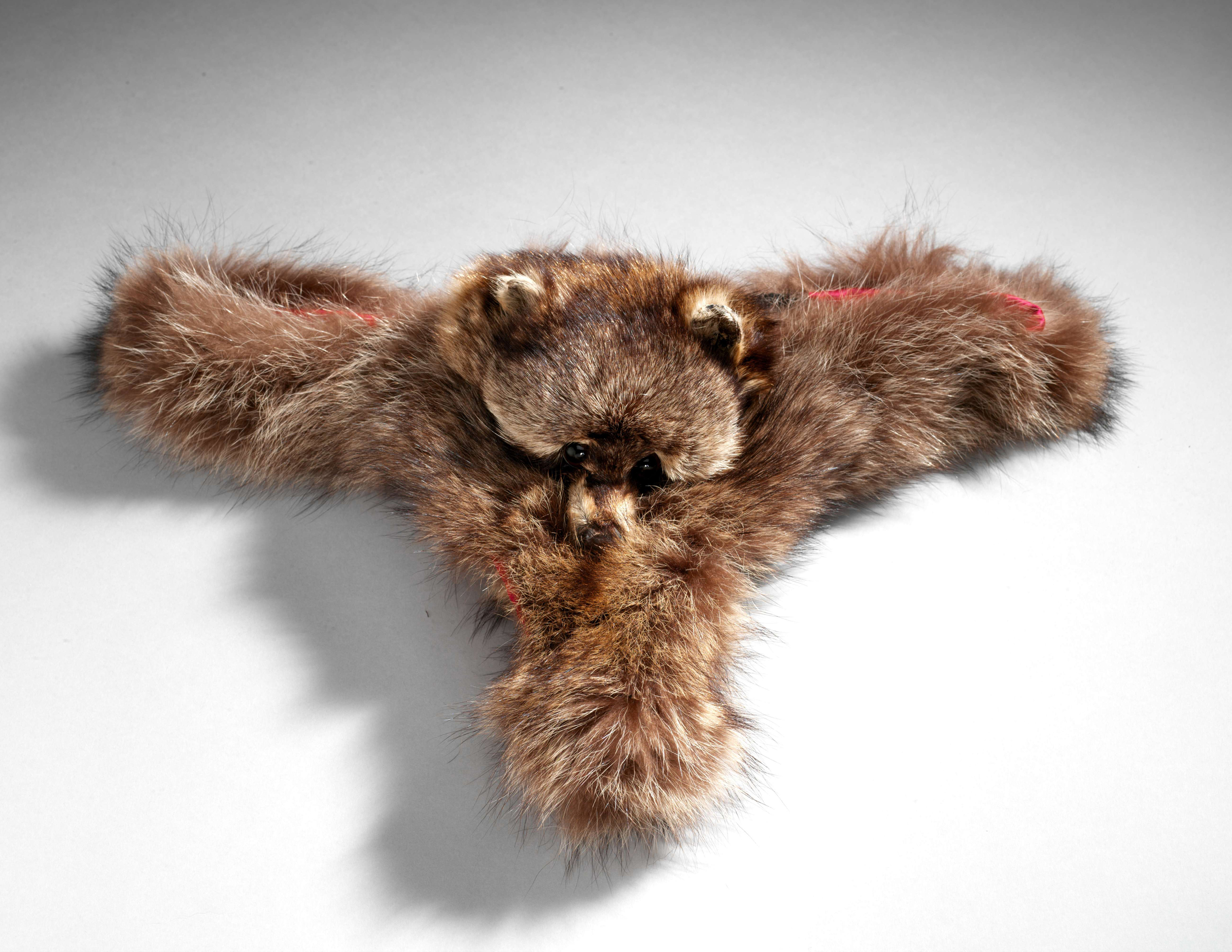The photo depicts a textured, fuzzy object resembling a furred creature, positioned against a white backdrop. The creature, which melds features of both a raccoon and a bear, exhibits a T-shaped layout with outstretched wings or arms. Its fur is a blend of dark brown, light brown, and hints of white, creating a rich and varied texture. Central to the image is the creature's round head, complete with beady black eyes, a small snout, and round ears trimmed in whitish fur. The eyes and snout exude an upward-facing, expressive demeanor. A distinctive red stripe runs horizontally across the top, above the outstretched wings. The creature's body extends downward in a triangular form, with a mix of brown and white fur seamlessly blending into the whole piece. The composition of the image and the creature's seemingly expressive face create a whimsical, yet enigmatic appearance.